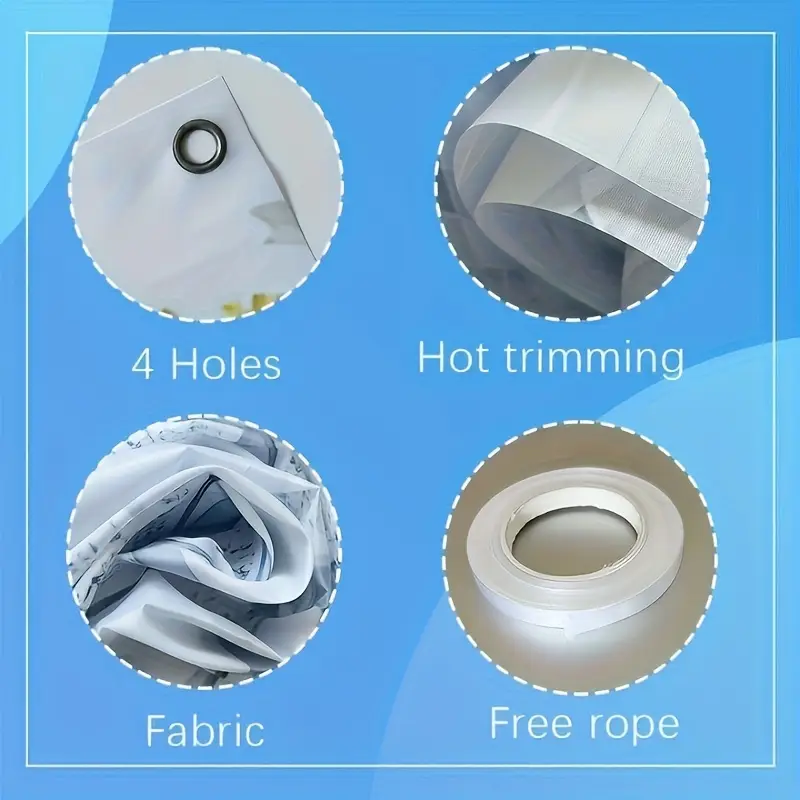The image depicts a blue square background, slightly taller than it is wide, with a thin white border. Inside the border are four circles, outlined in white dashes. Each circle contains an image and is accompanied by a descriptive caption below it in white text. 

In the upper left circle, labeled "Four Holes," there is a white piece of material featuring a silver grommet. The upper right circle, labeled "Hot Trimming," displays white plastic sheets folded over one another. The bottom left circle, marked "Fabric," shows neatly folded black and white fabric. The bottom right circle, captioned "Free Rope," contains a coil of white material resembling tape or ribbon.